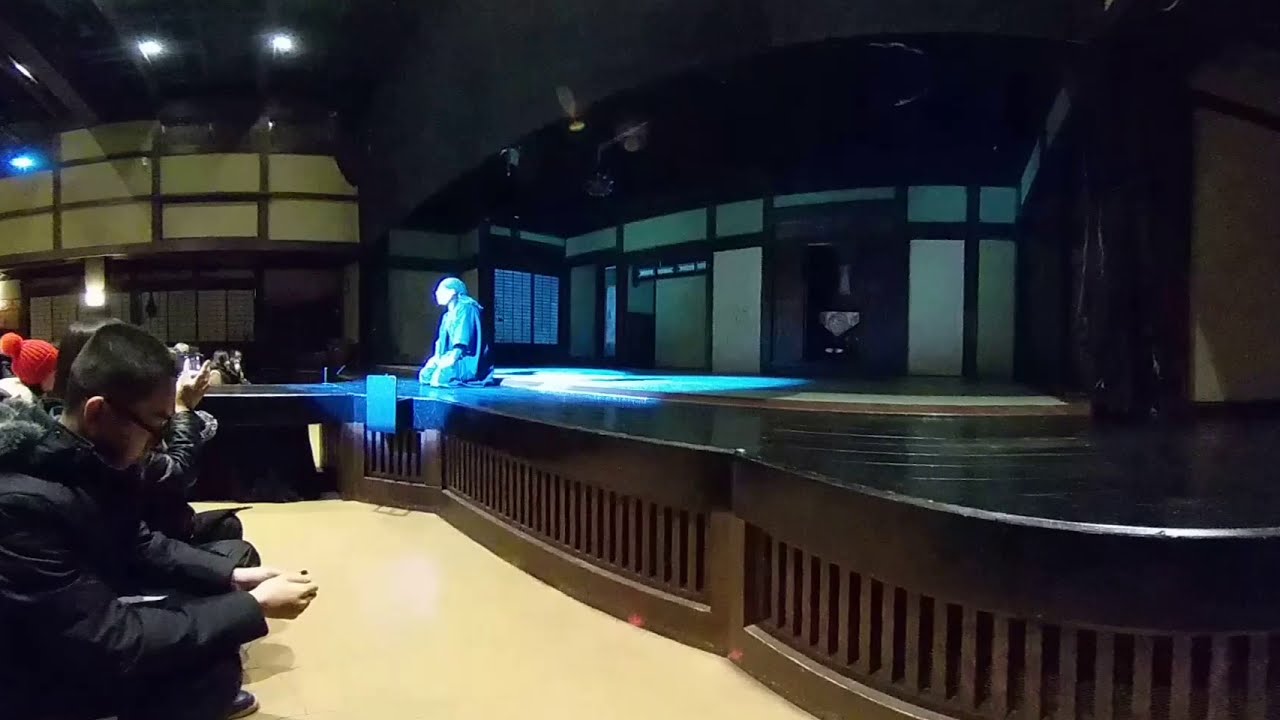In the image, a performance is taking place on a stage within an auditorium. The performer, dressed in all black with a head covering, is kneeling with both knees on the dark brown and black stage, illuminated by bright white and blue lights shining from the ceiling. Surrounding the stage, the walls are a mix of tan and brown, and a window with shades can be seen in the background. The audience, seated on tan flooring, appears partially disengaged, with many viewers focusing on their phones. Notably, a young male in the front row, wearing glasses and a black jacket with a gray fur-lined hood, looks downward. Next to him, a person in a leather jacket captures the scene with their phone. Another individual, identifiable by their red beanie, is also in the audience. The auditorium's black ceiling features multiple lights beaming down, enhancing the scene's visibility.